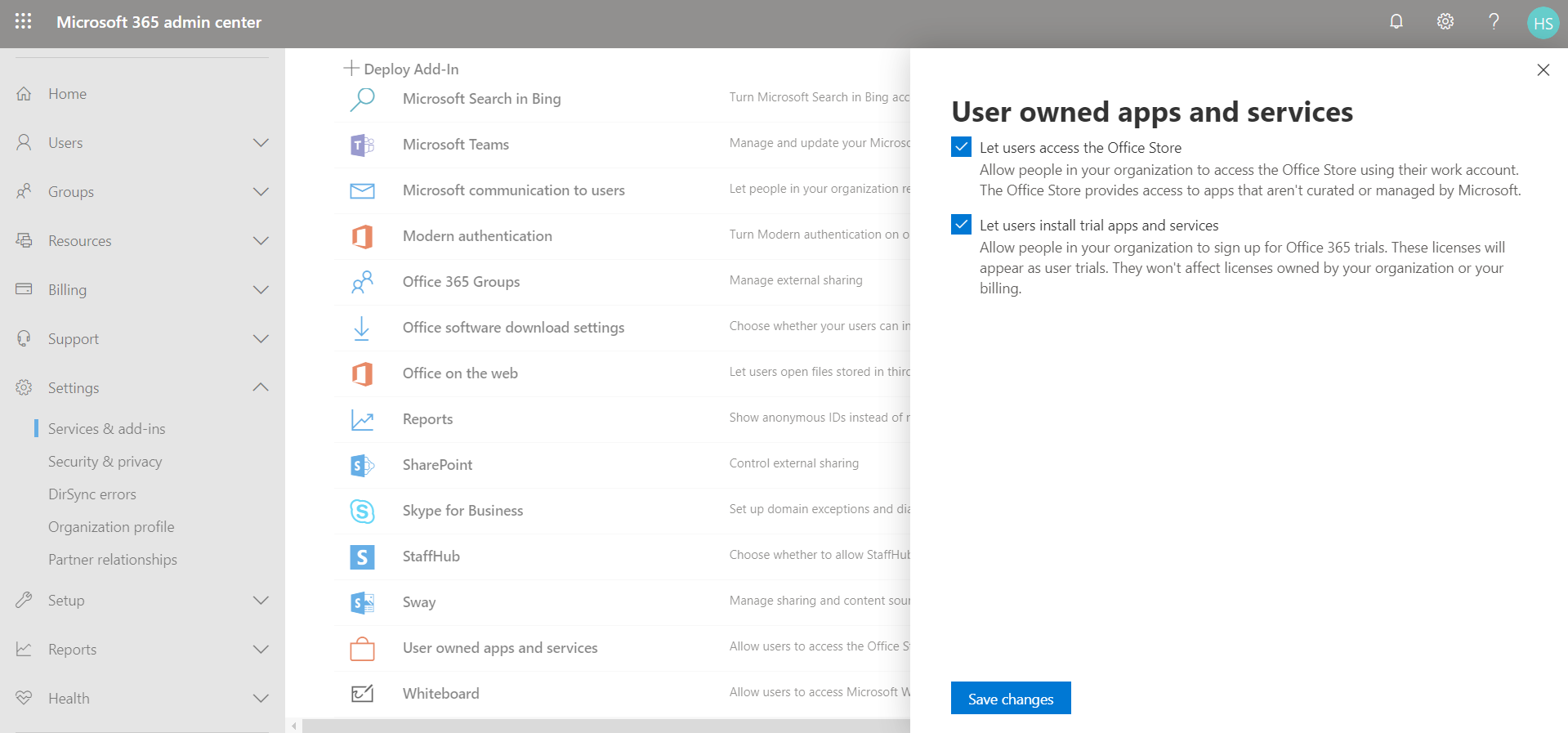**Caption:**

This screenshot captures the Microsoft 365 Admin Center interface, divided into three distinct panels. The leftmost panel, which is grayed out, features a vertical list of tabs: Home, Users, Groups, Resources, Billing, Support, Settings, Setup, Reports, and Health. Notably, the Settings tab is expanded, revealing five sub-tabs. The "Services & Add-ins" sub-tab is selected, indicated by a blue vertical highlight.

In the central panel, a "Deploy Add-in" button sits prominently at the top, urging administrators to add new functionalities. Below it is an extensive list of service settings, starting with "Microsoft Search in Bing," followed by "Microsoft Teams," "Microsoft Communication to Users," "Modern Authentication," "Office 365 Groups," "Office Software Download Settings," "Office on the Web," among others.

The rightmost panel is partially visible, displaying sections related to user management. Here, two checked options indicate features under "User-owned Apps and Services," suggesting active configurations or permissions.

The detailed layout provides a comprehensive view for administrators to manage services and settings within the Microsoft 365 ecosystem efficiently.